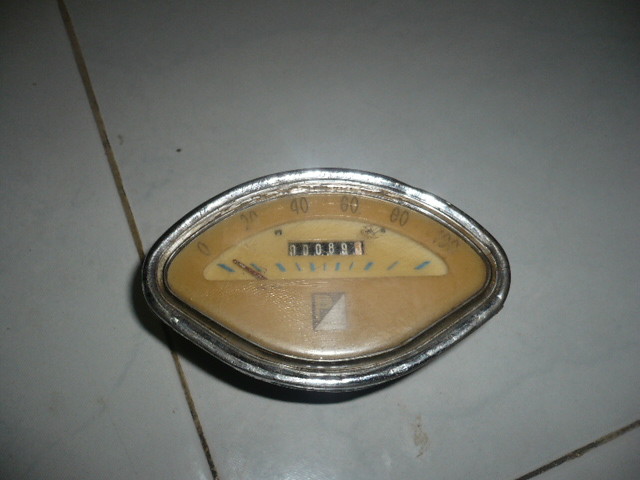The photograph captures a vintage speedometer or odometer from an old car, meticulously displayed indoors. The image is taken from an overhead perspective, focusing down on the instrument. The speedometer is positioned on a white tile surface, with distinct brown grout lining the spaces between the tiles. The speedometer itself is a flattened oval shape, encased in a shiny chrome frame. Its face is a muted tan color. The top arc of the speedometer displays the numbers 0, 20, 40, 60, 80, and 100, marked in clean, legible text. Thin blue dashes run along the center, guiding the progress of a red needle that points to the current speed. Prominently featured in the center of the speedometer is the odometer, which indicates a reading of 000893, suggesting minimal use. The overall composition offers a nostalgic glimpse into automotive history, accentuated by the contrasting modern and vintage elements.